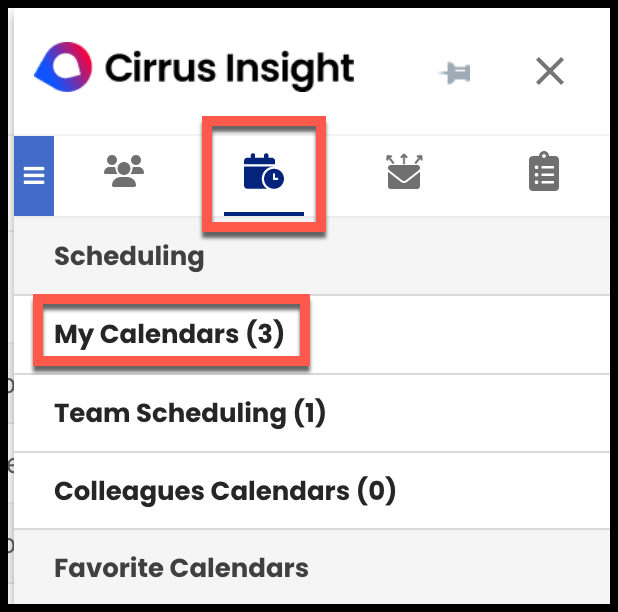The image depicts a screenshot of a section from an online application. The main focus is a square window framed by a thick black border. Inside this frame, the window has a white background that is partitioned into rows separated by gray horizontal lines. In the upper left corner, there is a circular logo with a pointed left side, featuring a dual color scheme of blue and red. Adjacent to the logo, black text reads "Cirrus Insight."

Directly below the logo, there are several icons, one of which is highlighted with a red square; this icon is blue and resembles a clock, suggesting it denotes time or scheduling. Below this icon, text appears in gray. The primary content consists of five rows, each labeled in gray text. The top row reads "Scheduling," and the rows below it read "My Calendars." The "My Calendars" row is distinctly highlighted in an orange rectangle.